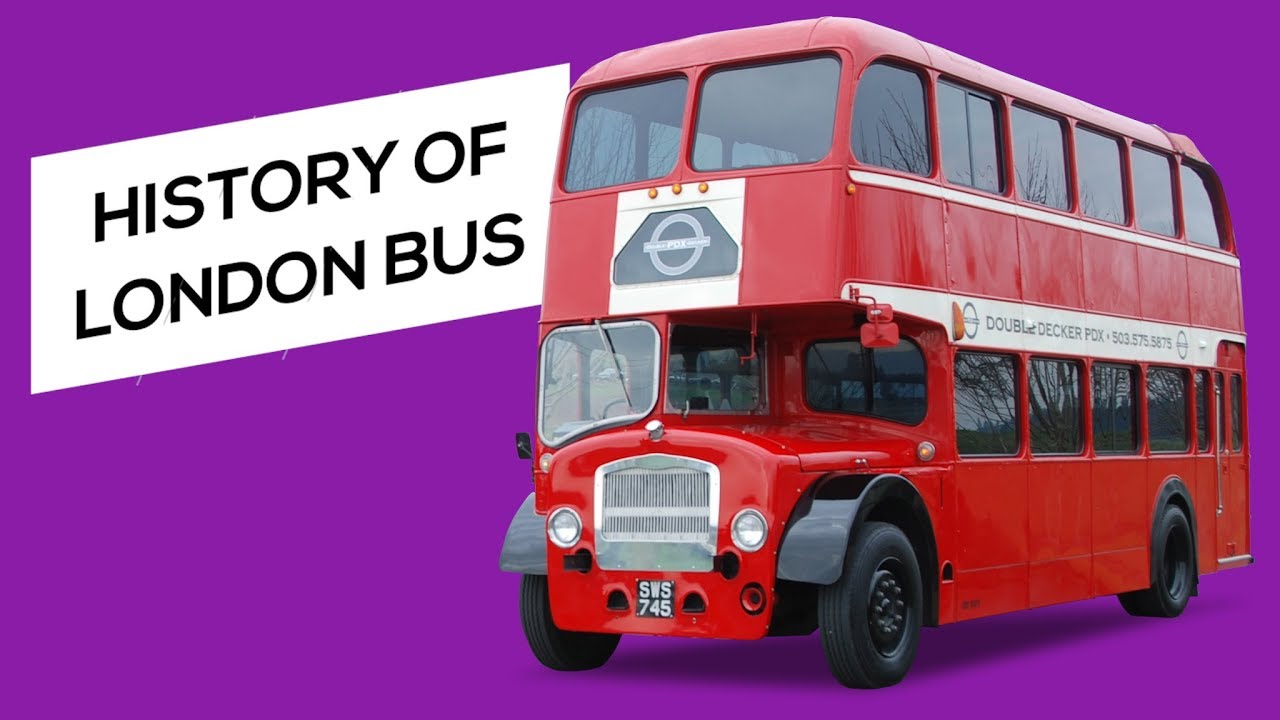The image features a well-crafted graphic with a vibrant purple background. On the left side, there is a prominent white rectangular banner bearing the text "History of London Bus" in bold black letters. Dominating the right side of the graphic is a traditional, eye-catching red double-decker bus with a license plate that reads "SWS 745." The bus, characterized by its two stories and multiple windows, includes a text inscription on its side reading "Double-Decker PDK" and a visible phone number "503-575-5875." The bus is depicted with clarity, emphasizing its iconic and towering structure, typical of the famous London buses. This image serves as an informative visual, likely promoting a program or exhibit dedicated to the historical significance of London's double-decker buses.